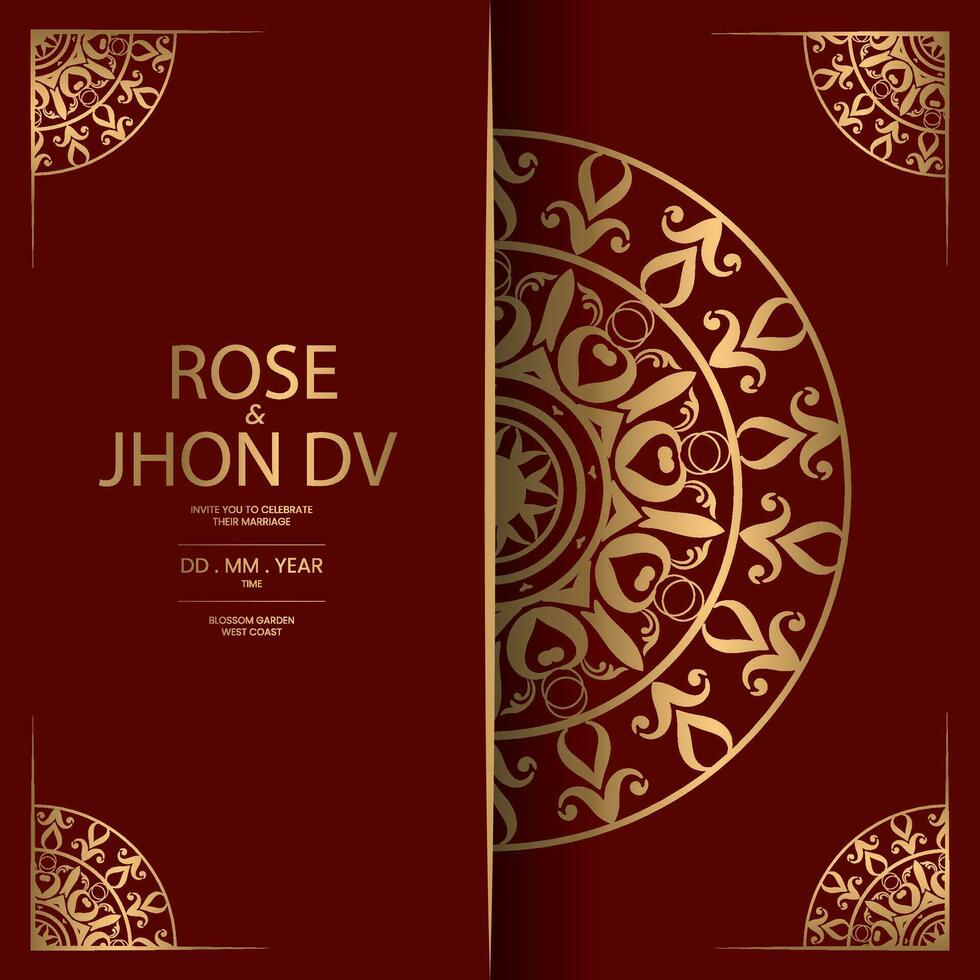This image depicts an opulent, digitally synthesized wedding invitation with a rich, burgundy red background adorned with intricate gold designs. At the center of the image runs a vertical line, thicker in the middle and tapering towards the top and bottom. To the left of this center line, prominently written in gold, are the names "Rose and John D.V." inviting guests to their marriage. Directly below, in smaller gold text, are the words "Invite You to Celebrate Their Marriage," followed by placeholders "DD.MM.Year" and "Time," and then "Blossom Garden, West Coast." On the right side, connected to the central line, is the right half of a mandala-like circle rendered in delicate gold patterns, allowing the burgundy background to show through. Each corner of the square image features a quarter of a similar mandala design, intricately spaced from the edges, enhancing the ornate and formal appeal of the invitation.